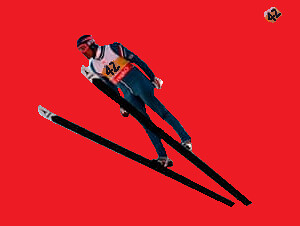The image depicts a ski jumper mid-flight against a solid red background. The athlete is fully airborne, leaning forward over a pair of skis that form a narrow V-shape, with the tips pointing outward. He is dressed in a tight, dark blue ski suit with matching sleeves and pants. Over the suit, he wears a white bib featuring the number 42, situated above an amber and red stripe across his diaphragm. The ski jumper's attire includes a black helmet and protective goggles. The skis are predominantly black, with the top six inches white, adorned with a black design. Additionally, the number 42 is prominently displayed in black lettering in the upper right corner of the image.